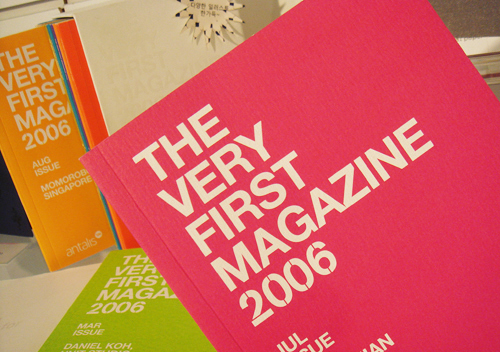The image captures a vivid and colorful arrangement of several magazines titled "The Very First Magazine, 2006." Dominating the foreground, a thin, hardcover booklet with a pinkish-red cover, bearing the white, left-justified text "The Very First Magazine, 2006" in separate lines, prominently displays the July issue. To its sides, other issues in various hues—such as the lime-colored March issue and the orange-covered August issue—are partially visible, some housed in a magazine container. Additionally, other magazines with colors like green, light blue, dark blue, yellow, and white are scattered and angled towards the left, casting delicate shadows onto a white surface beneath them. The collective array creates a vibrant and engaging visual tapestry, emphasizing the uniform title across diverse monthly issues.